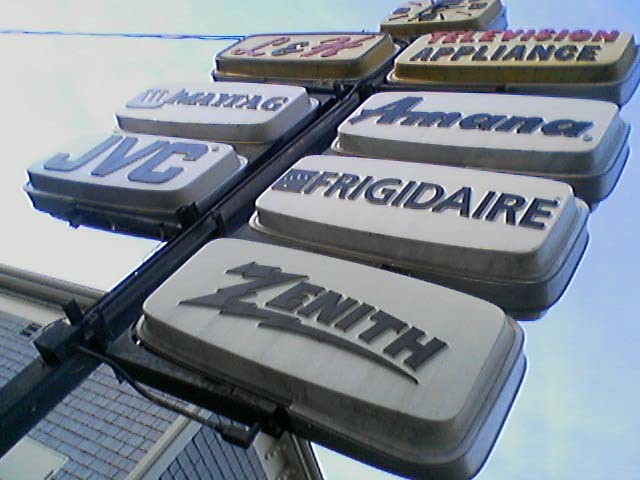The photograph captures a nostalgic scene from the ground looking up at an old-fashioned sign in front of an appliance store, likely from the 1970s. The sign is mounted on a sturdy black metal pole, with visible electric wires extending from a transformer, supplying power to the various sections of the sign. At the very top of the sign, there's a clock face indicating the time. 

The sign prominently features "L&H" in bold letters, followed by "Television" and "Appliance," designating it as the L&H Television and Appliance Store. Below this header, several well-known brand logos are displayed, including Maytag, Frigidaire, JVC, and Zenith, along with the Maytag and MANA logos.

In the backdrop, there is a building clad in gray asbestos tiles, crowned with a white gutter along its top edge. Above, an electrical wire stretches across the sky, adding to the vintage ambiance of the image. The clear sky highlights the distinct, aged aesthetic of both the sign and the architecture, evoking a sense of time long past.